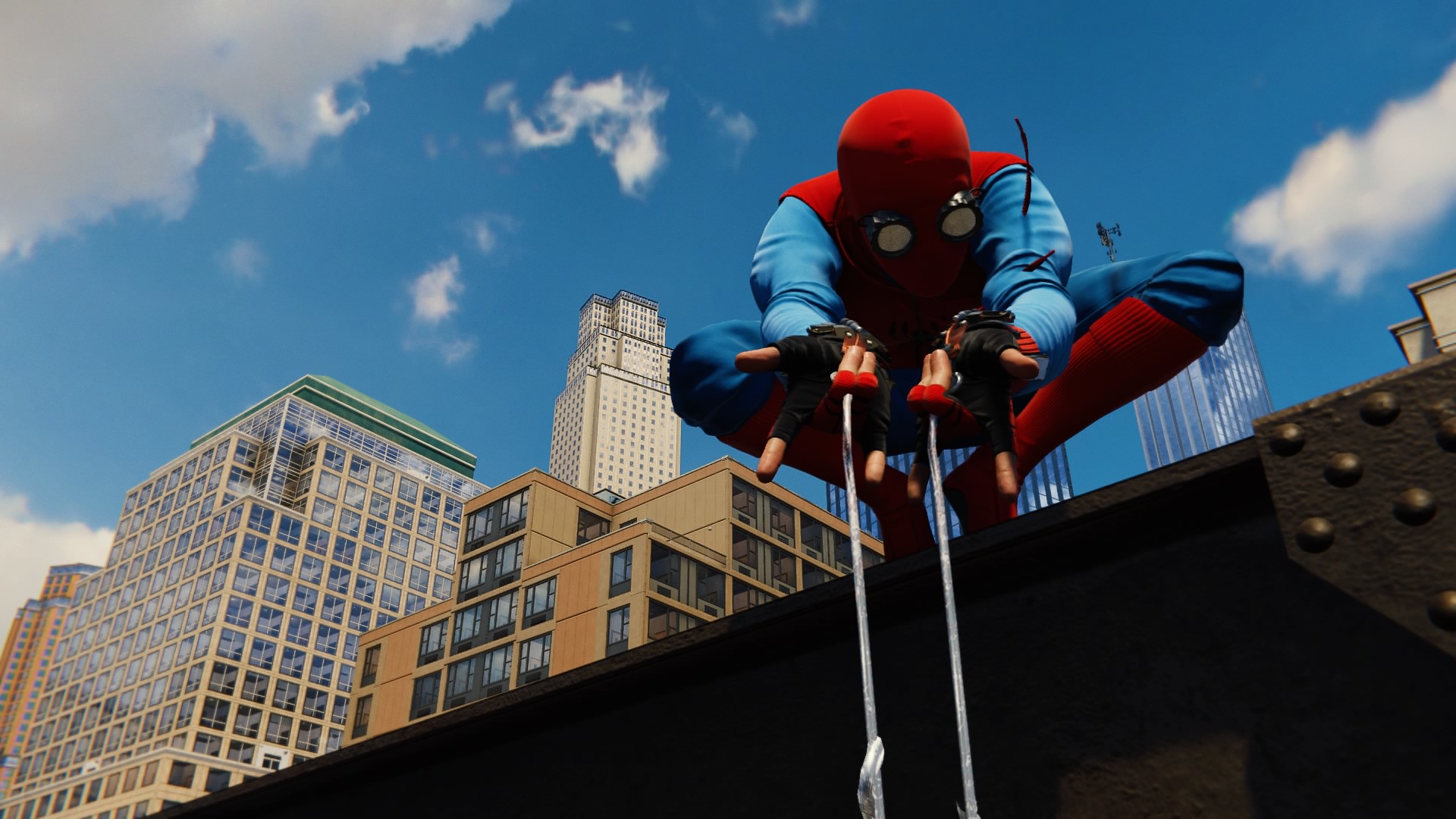This image, likely from a video game, showcases an individual dressed in a very budget Spider-Man costume against the New York skyline. The person, approximately five and a half feet tall but crouched, is perched on a steel girder with a clear day sky and a few clouds in the background. The costume features a red mask with black goggles outlined in white, a red vest over a blue sweater, blue sweatpants, red boots, and black fingerless gloves with some red accents. The individual is shooting crystalline, slimy-looking webs from their hands, which hang straight down. The skyline features a variety of skyscrapers, including a very tall beige one and others in shades of beige, cream, tan, and even a blue building on the right side. The buildings and girder are glimpsed from a low angle, making the scene feel dynamic and action-packed.